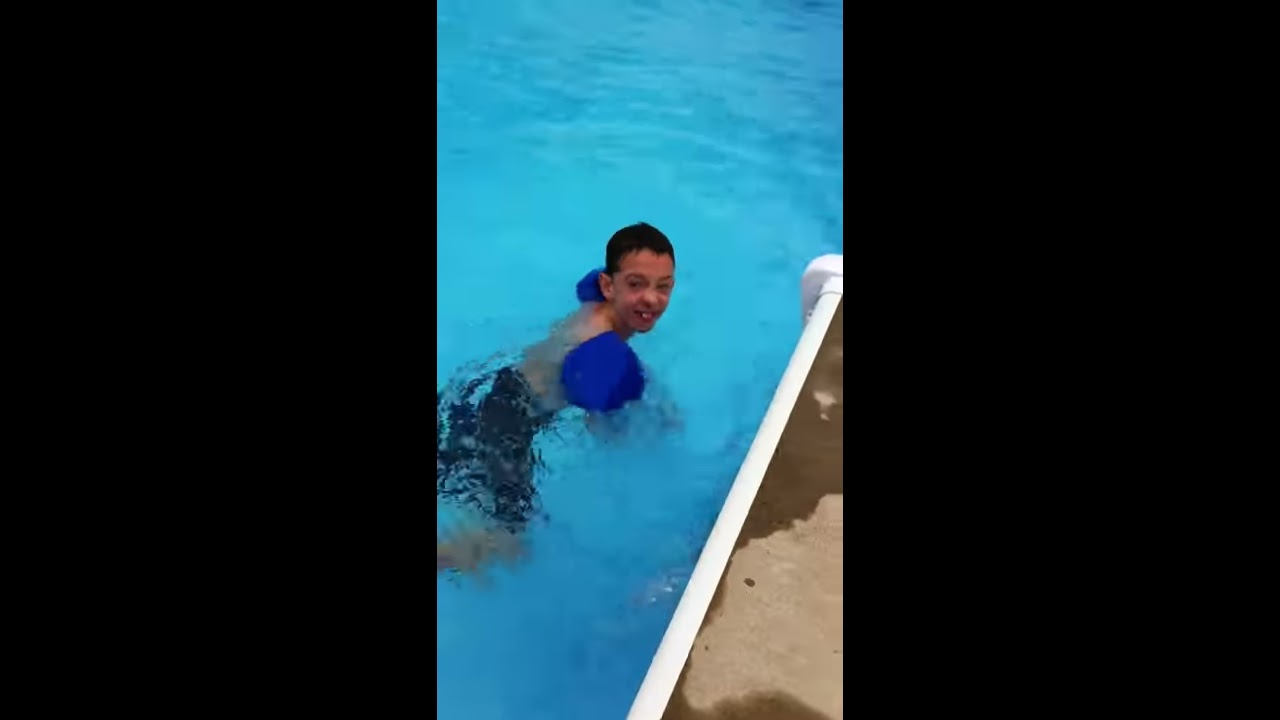In the center of a bordered image with thick black margins on the left and right, a young boy of about 10 to 12 years old is seen enjoying himself in a swimming pool. The vibrant, crystal-clear blue water contrasts with the white-edged cement pool deck visible in the lower right corner of the picture, which appears partially wet and dry. The boy, of Caucasian descent, has short, dark brown or black wet hair and wears dark blue or black swim trunks. Large blue water wings are strapped to his upper arms, aiding his buoyancy as he swims. With a goofy smile, he looks back over his shoulder at the person taking the picture, his face scrunched up in a playful expression that exudes joy and amusement. The angle of the pool runs diagonally from the midline of the right side to the bottom, emphasizing the dynamic setting of this lively moment.